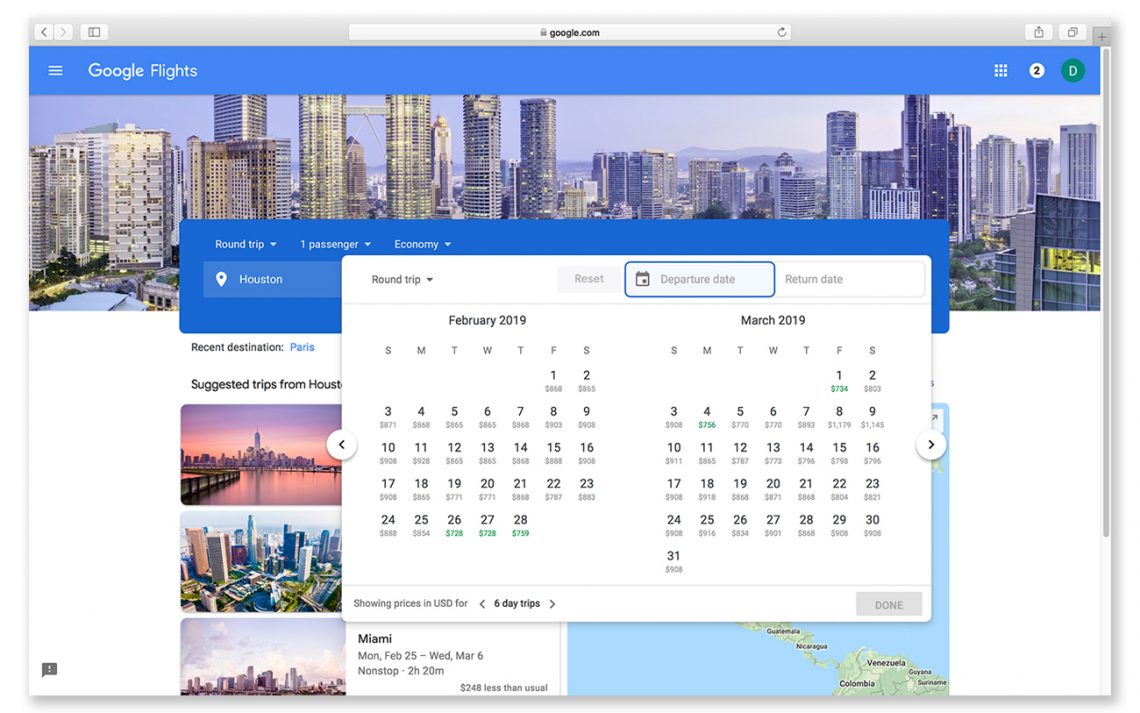The image depicts a flight booking section of a website featuring a user interface with various navigational elements. At the very top, there is a gray border containing 'back' and 'forward' buttons on the left corner, an address bar in the center displaying "google.com" accompanied by a refresh icon on the right. Beneath this, a blue border showcases three horizontal white lines indicating a menu for more options, next to the label "Google Flights." There is a grid icon and a green circle with the letter "D" on the far right.

Below this toolbar, an image highlights skyscrapers and a city skyline. Directly under the image, a blue box states "roundtrip, one passenger, economy, Houston" with a pop-up box specifying "roundtrip" and a blue-highlighted "departure date" box. The calendar displays months February 2019 and March 2019, showing various pricing options. Additionally, there are other images depicting skylines of different cities, providing further visual context to the booking options.